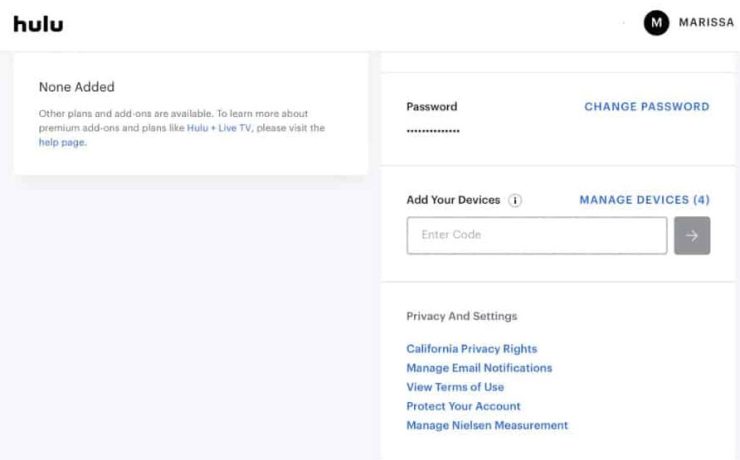Here is a cleaned-up and detailed caption for the image described:

"A screenshot from the desktop version of the Hulu website. At the top, there's a white border with the Hulu logo in black located in the upper left corner. On the upper right corner, there's a black circle containing a white 'M', which represents the initial of the user, Marissa, whose name appears to the right of the image. On the left side of the screen, there's a gray box with a white section inside it indicating 'None added' for additional subscriptions, accompanied by a message mentioning that other plans and add-ons are available. This suggests that Marissa has not opted for any extra channels or services like Showtime or Starz. To the right of this section, there's a series of white boxes. The first box concerns the user's password, featuring a blue button labeled 'Change Password' on its right side. Below this, there's a section for adding devices that can access the account, with a box provided for entering the necessary code to add these devices. Further down, the screenshot includes the 'Privacy and Settings' section, detailing options for user privacy and account settings management."